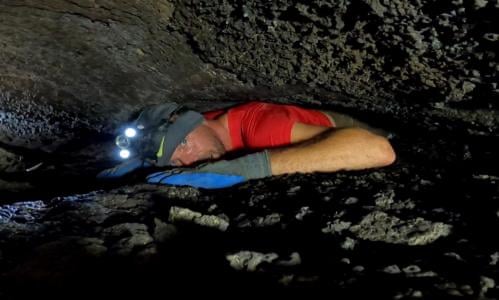The image is a color photograph in landscape orientation, capturing a man, approximately 30 years old, engaged in spelunking. He is navigating a narrow passage in a cave, squeezed tightly between two large, rough, and jagged rock formations. The man is depicted from the top of his head to about mid-waist. His left arm is folded in front of his face, resting on a rock with a gray glove that has a blue palm. He is wearing a short-sleeved red shirt and a dark gray cap with a headlamp featuring two round white bulbs, shining light toward the camera. His blue eyes are visible as he faces the camera, with his expression suggesting either effort or focus. The cave around him consists of dark gray rocks with striations of greenish-olive colors and black hues, with the rocks appearing darker near the bottom and lighter near the top, possibly due to the lighting. The scene is illuminated primarily by the headlamp he is wearing and an additional light source from the camera. The background is almost pitch black, making it difficult to discern any further details beyond the man.